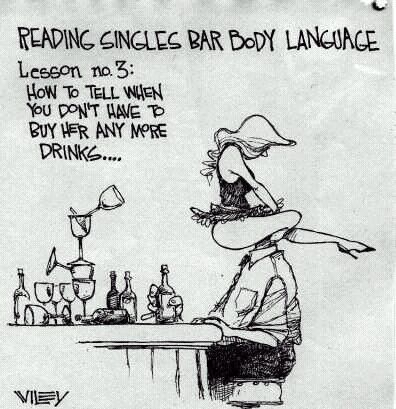The image is a humorous black-and-white cartoon featuring a bar setting. At the center of the illustration, a man is seated at a bar counter cluttered with numerous empty drinking glasses and bottles. A woman with long, presumably blonde hair, based on the lack of shading that suggests light color, is depicted wearing lingerie and high heels. She is suggestively positioned atop the man's shoulders, with her legs wrapped around his head and her left leg extended outward. The cartoon's caption reads, "Reading singles bar body language. Lesson number three: How to tell when you don't have to buy her any more drinks." The artist's signature, Wiley, is visible in the lower left corner. The background is a light hue, potentially green or gray, enhancing the monochromatic scheme of the illustration.